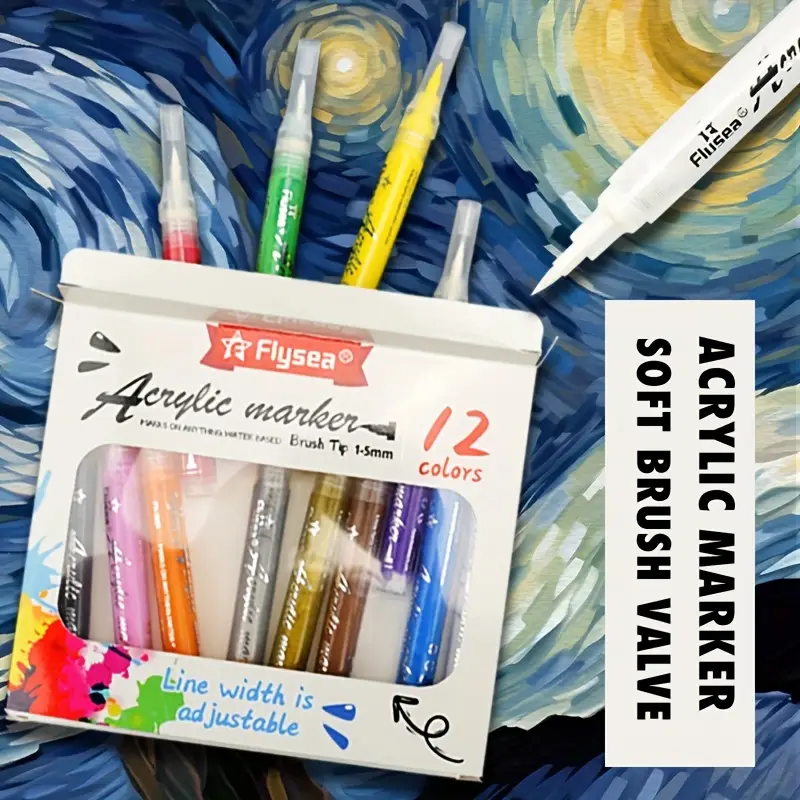This image features a box of 12 vibrant acrylic markers by the brand Flicy, identifiable by its red and white logo. The markers, varying in colors including red, green, yellow, purple, and white, are positioned on top of a painting reminiscent of Van Gogh's style with swirling dark and light blues and yellows. On the right side of the image, there is a label within a white box containing black text that reads "Acrylic Marker Soft Brush Valve." On the left side of the box, another text states "Acrylic Marker 12 Colors." The box also has a small plastic window showcasing the array of colors inside. The painting beneath the markers evokes the night sky theme iconic in impressionist art, with swirling patterns and a luminescent presence, contributing to an overall dynamic and textured background.